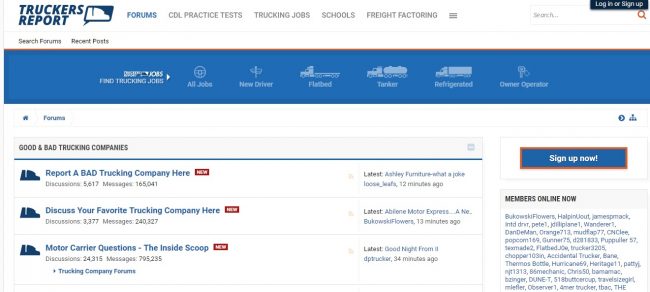This is a detailed and descriptive caption for the screenshot from the Trucker's Report webpage:

---

The screenshot captures the Trucker's Report webpage, featuring a predominantly white background with a distinctive blue rectangular section located in the upper middle of the page. On the top left, the page displays the Trucker's Report logo, which consists of a blue quotation bubble encompassing a white truck silhouette. Adjacent to the logo are several navigation options: FORUMS, which is currently selected and highlighted in blue, as well as CDL Practice Tests, Trucking Jobs, Schools, Freight Factoring, and a menu represented by three horizontal gray lines.

To the right of these navigation options is a search bar equipped with an orange magnifying glass icon. Above this search bar, there's a prominently placed action button labeled "Log In or Sign Up," featuring white text on a dark blue background.

Below the navigation bar is the FORUMS section, which begins with two available tabs: "Search FORUMS" and "Recent Posts." The header of the FORUMS portion stands out with a blue background and contains initial descriptive text, including "Find Trucking Jobs," followed by six icon-based options. These options include:

1. **ALL JOBS** - represented by a circular symbol resembling an eye.
2. **NEW DRIVER** - illustrated by a road sign-like icon pointing left.
3. **FLATBED** - depicted with an image of a flatbed truck facing left.
4. **TANKER** - symbolized by an oil tanker truck icon facing left.
5. **REFRIGERATED** - shown as a standard semi-truck logo.
6. **OWNER OPERATOR** - represented by an image of a single key with a keyring.

The main body of the FORUMS section comprises a table displaying various discussion boards, each beginning with the Trucker's Report logo followed by the board's title. The featured boards include:
- **REPORT A BAD TRUCKING COMPANY** - marked with a red "NEW" box.
- **DISCUSS YOUR FAVORITE TRUCKING COMPANY** - also accompanied by a red "NEW" box.
- **MOTOR CARRIER QUESTIONS** - similarly marked with a red "NEW" box.

Each board entry is separated by thin gray dividing lines, with the latest post information listed in the right column for each board.

To the right of this table section, there is a prominent "SIGN UP NOW" button with an orange outline, blue fill, and white text. Below this button, there is a box displaying the usernames of currently online members, which are arrayed in approximately ten rows with three to four generic usernames in each row.